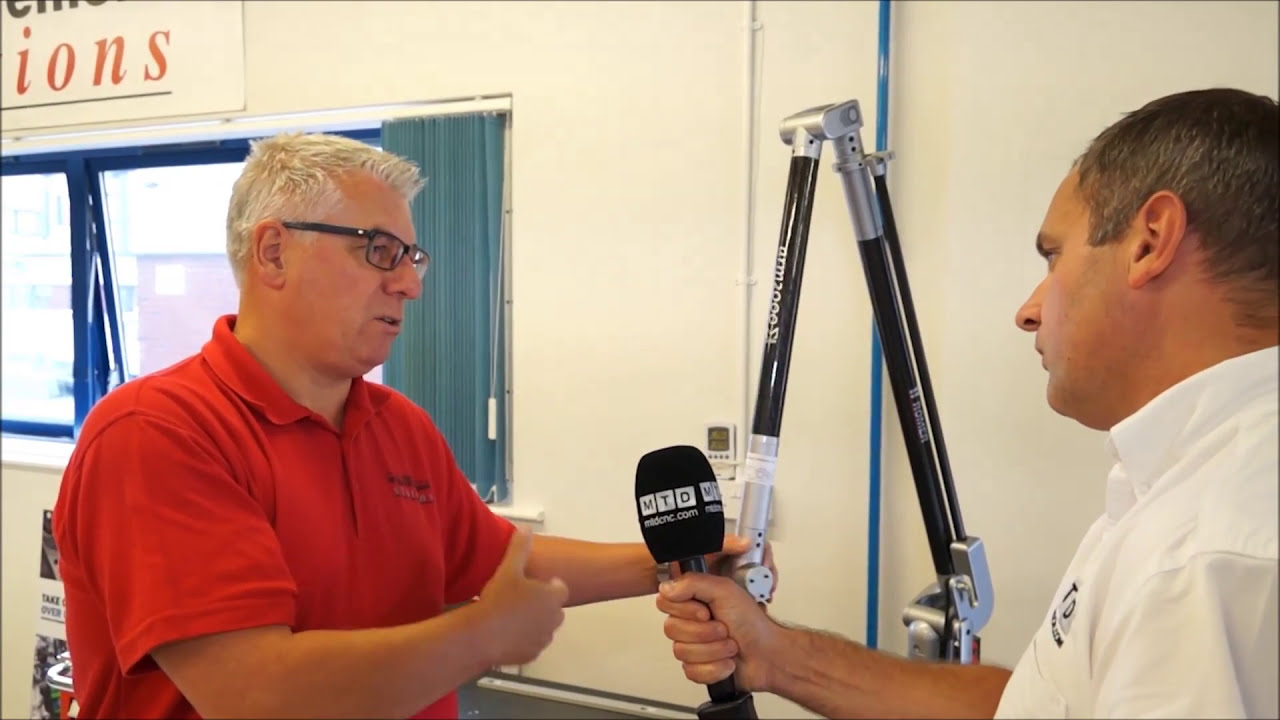The photograph captures a detailed indoor scene featuring two men in an apparent interview setting, likely within an office. On the right side stands a man with short dark hair, dressed in a white short-sleeved collared shirt adorned with black lettering on the left chest. He is holding a black microphone with white print that reads "mtdcnc.com" in uppercase letters. Adjacent to this microphone, close to the white wall, is a black and stainless steel mechanical arm. The man appears to be in his 40s, standing from mid-chest up with his right arm extended as he conducts the interview.

On the left stands the interviewee, a heavier set man with short, slightly spiked white hair and black-rimmed glasses. He is wearing a red polo shirt featuring black lettering on the left chest. This man stands in front of a full-length window trimmed in dark blue, with turquoise-colored curtains partially slid to the side. His right arm is crossed in front of him, while his left arm is extended forward, grasping a boom mic. Above his head, there is a sign with red lettering that partially reads "IONS." The background also includes a thin pinstripe black border around the white wall, adding to the meticulous detail of the scene.